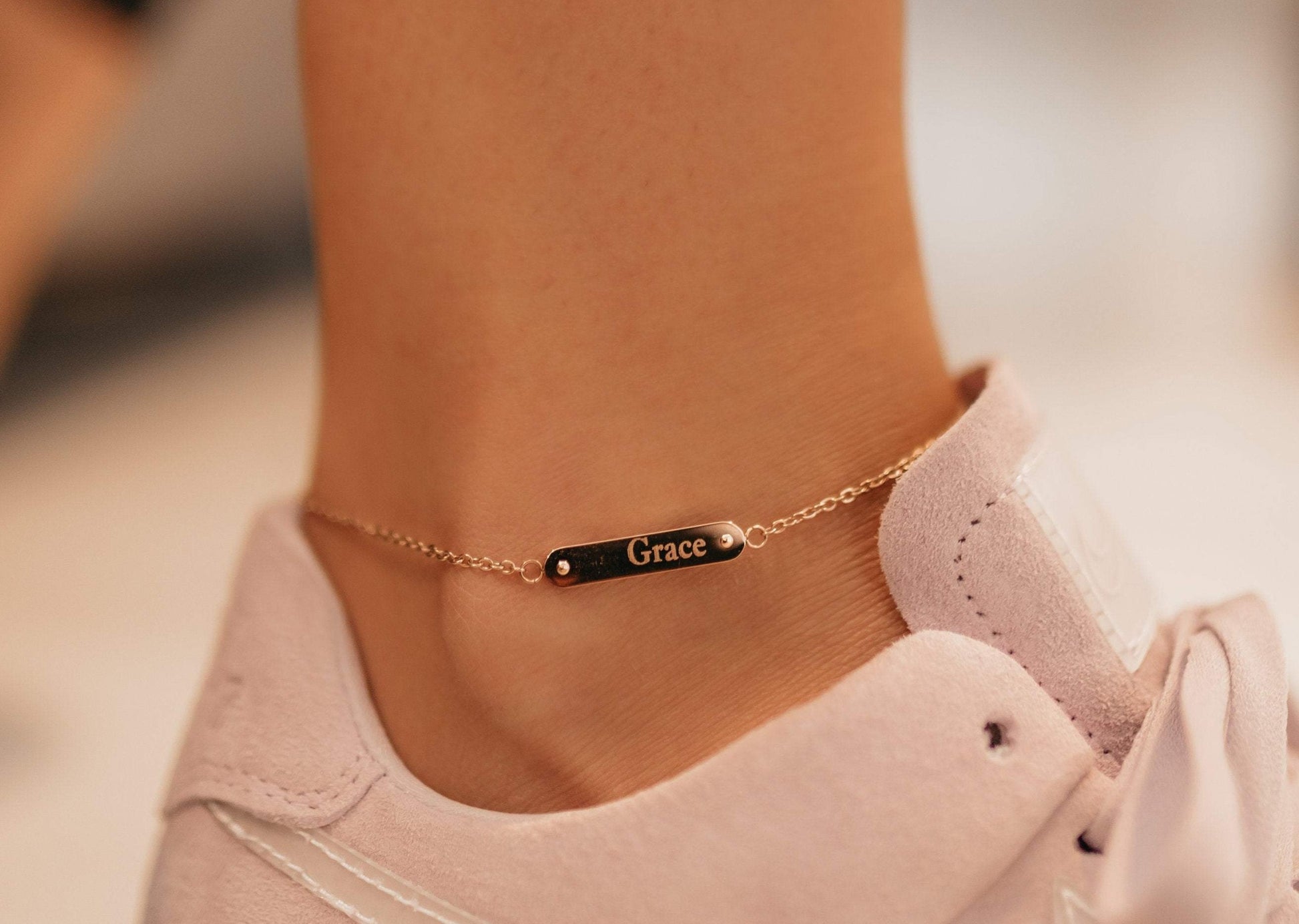The photograph is a close-up of a woman's ankle adorned with an anklet. The anklet is a delicate gold chain with a rectangular nameplate inscribed with the name "Grace," written with a capital "G" followed by lowercase "r-a-c-e," positioned off to the right. The woman's skin is light, and she is wearing a well-worn, low-cut suede shoe in an off-white color, revealing her ankle. The shoe has thick laces that do not go all the way up to the last hole, leaving the top hole undone. The background of the image is blurry, with hints of a white or off-white surface, possibly a carpet. This extreme close-up captures the forward foot, slightly stepping forward, offering a detailed view of the anklet and the shoe.